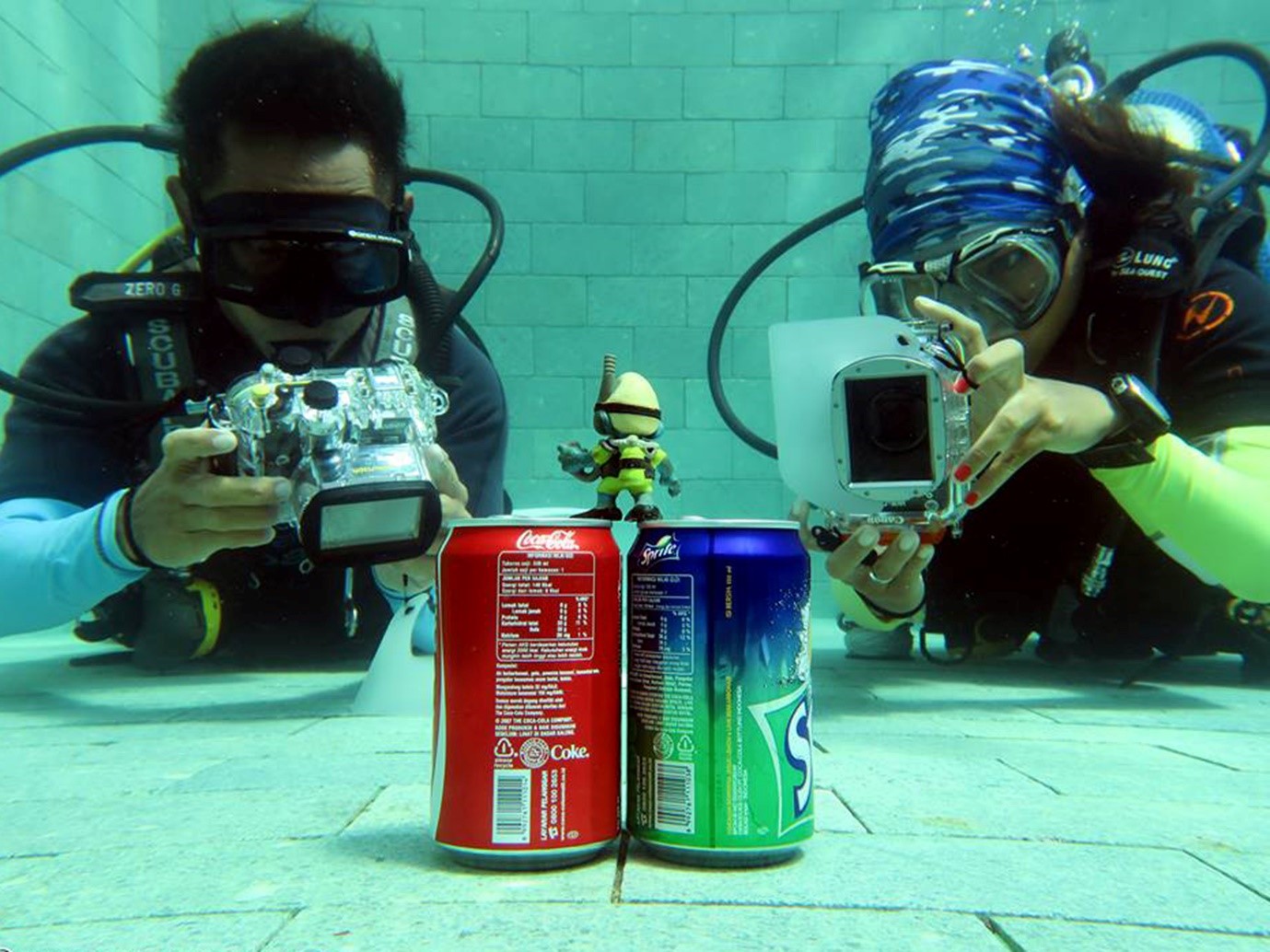A vibrant, full-color, staged photograph captures an underwater scene in a sunlit pool, showcasing a peculiar, yet amusing setup. The pool's blue-brick floor and walls provide the backdrop. Central to the composition are two aluminum soda cans – a red Coca-Cola can and a blue and green Sprite can – situated side by side, their backs facing the camera. Standing atop these cans is a small figurine reminiscent of an underwater alien, dressed in a suit with a mask and gun. 

In the foreground, two scuba divers lay on their stomachs, facing the cans with cameras in hand. On the left, a man with short black hair and black diving goggles wields a traditional waterproof underwater camera equipped with a protruding lens. On the right, a woman sporting a blue, camouflage-patterned bandana and nail polish, wears two-lens goggles and uses an iPad-like camera featuring a large front lens. She also has a watch on her left wrist. The clear visibility underwater hints at daytime natural lighting, contributing to the sharp details and vibrant colors of the scene.